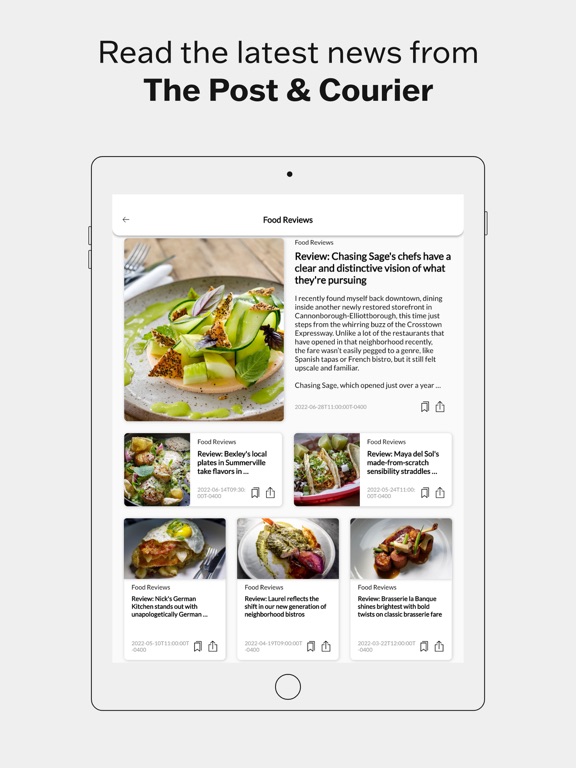**Detailed Descriptive Caption:**

The advertisement features a clean, white background with bold black lettering at the top that reads, "Read the latest news from The Post and Courier." Beneath this text, an image of a simulated iPad is displayed in portrait mode, showcasing a food review website. At the top of the iPad's screen, the title "Food Reviews" is prominently featured. Below this title, there is a tantalizing image of a meticulously prepared dish. To the right of the dish, bold text announces a review titled, "Chasing Sage's Chefs." The accompanying subtext highlights that "Chasing Sage's Chefs have a clear and distinctive vision of what they're pursuing." Further down the simulated iPad screen, smaller text from an article is visible but unreadable. Additional images of various food dishes are displayed lower on the page, each accompanied by headlines starting with "Review." One specific headline reads, "Review: Becky's Local Plants in Somerville, take flavors in," elucidating that the site offers detailed reviews of local culinary creations. This advertisement effectively showcases a vibrant, interactive food review section of The Post and Courier website.